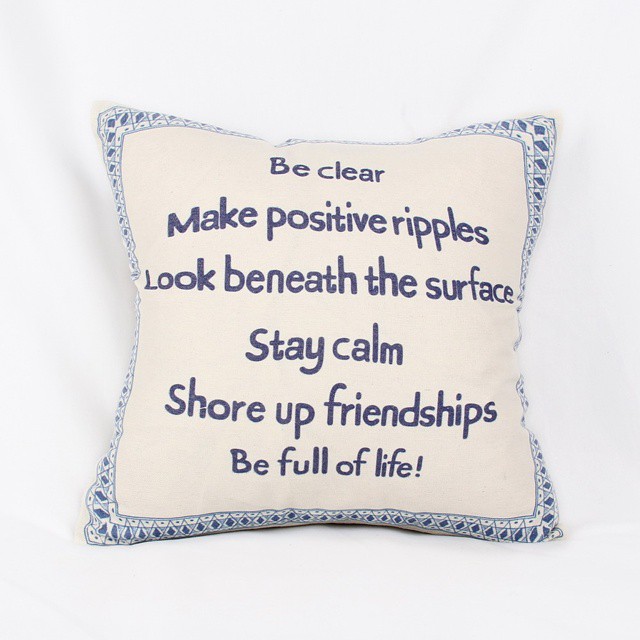The image depicts a square throw pillow resting on a slightly wrinkled white background, possibly a bed sheet or comforter. The pillow itself is a light pink or off-white color, enhanced with a distinct blue border. This blue border features a central line adorned with diamond shapes, flanked by inner and outer lines of polka dots. In the center of the pillow, blue text runs vertically, extending from the top to almost the bottom of the pillow, conveying the positive message: "Be clear, make positive ripples, look beneath the surface, stay calm, shore up friendships, be full of life!" The pillow appears plush and well-stuffed, giving it a rounded and fluffy appearance.